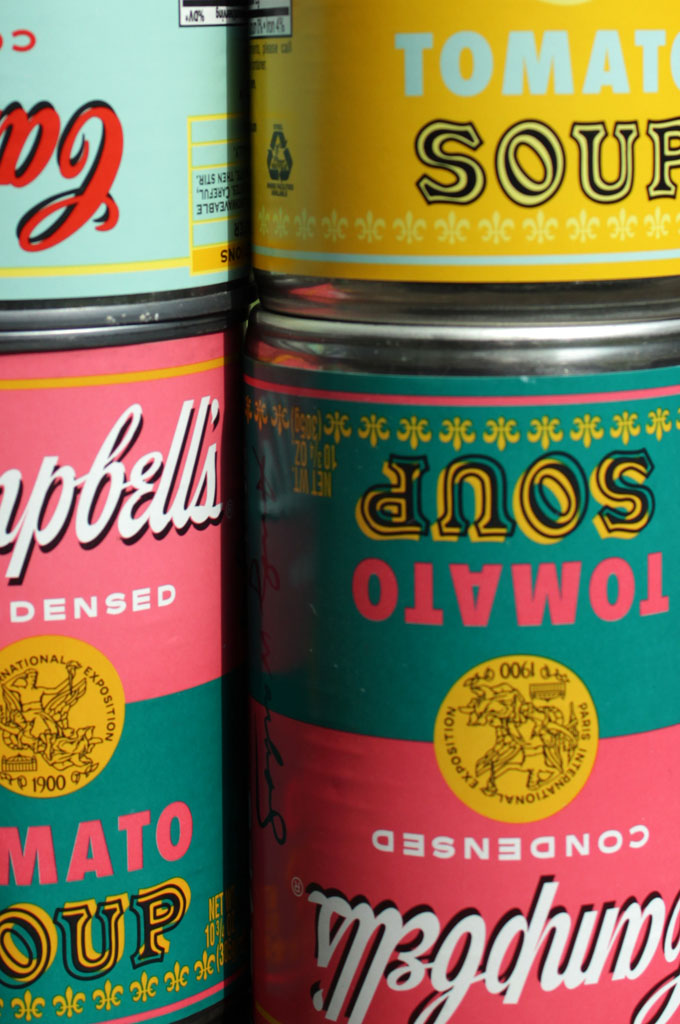The image displays four vividly colored Campbell's soup cans, arranged in a stacked formation of two cans per row. The topmost can is positioned upside down, revealing only the letters "CA" of the iconic Campbell's logo. This can features a light blue background complemented by yellow accents, with the Campbell's text elegantly written in red.

Beneath the top can is another intriguing soup can colored in a rich pink with teal accents. The partial logo visible reads "P B E L L" followed by an apostrophe and "s." Additionally, only the segment "densed" of the word "condensed" is visible under the Campbell's logo. This can is labeled "tomato soup."

Beside the described cans, another pair is stacked similarly, with the top can also upside down. The visual similarities in color and logos confirm that it is identical to its adjacent counterpart. The combination of these cans creates a colorful and symmetrical arrangement, drawing attention to the vibrant design and classic branding of Campbell's soup.